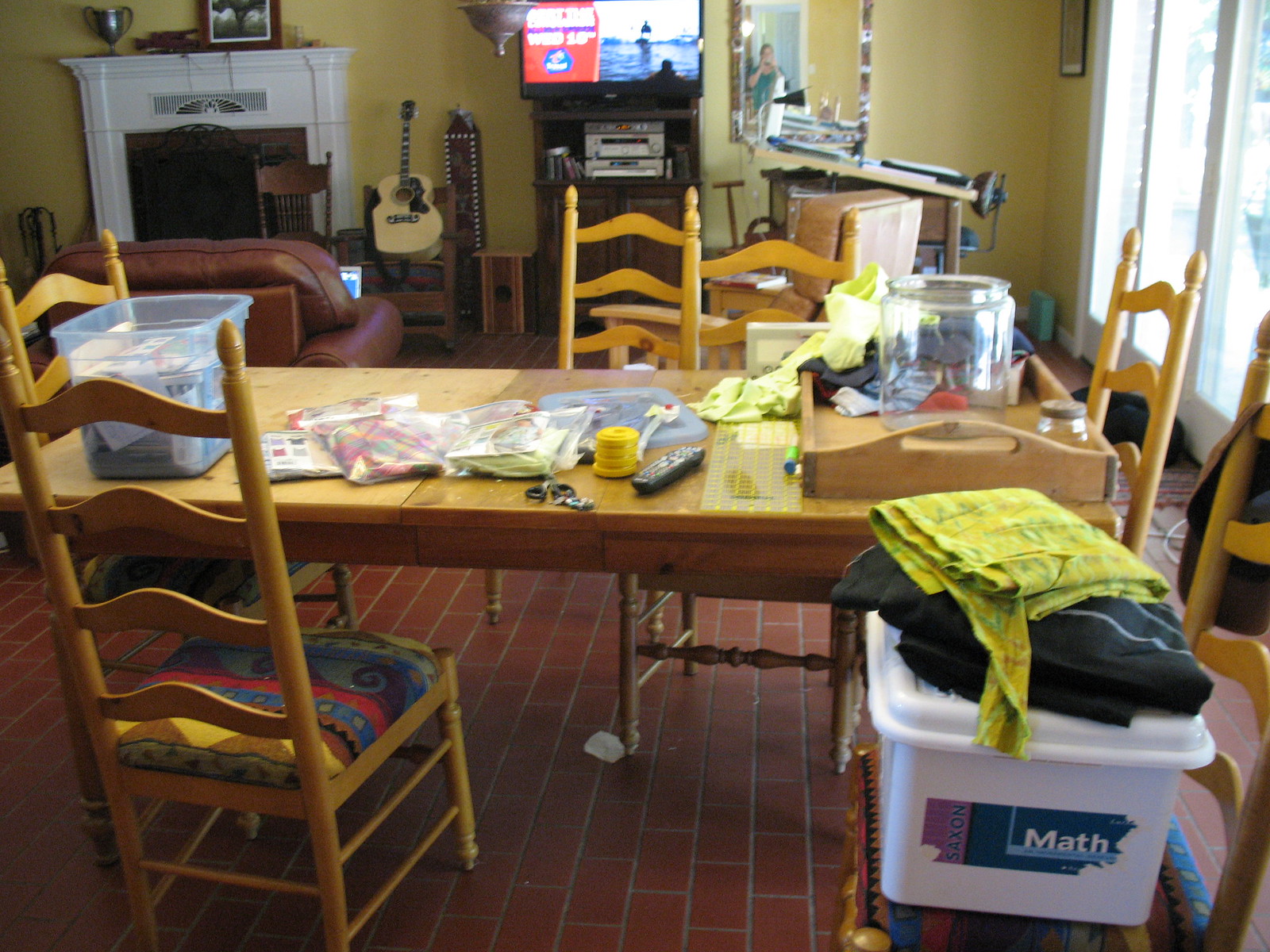A vibrant color photograph captures the cozy chaos of a cluttered living room. In the top left corner, a pristine white fireplace stands out, with a wooden chair positioned in front of it. To the right of the chair, a light brown guitar leans serenely. Dominating the foreground is a rectangular light brown table surrounded by assorted chairs. The table's surface is a medley of objects, including a large clear jar, a remote control, and an open pair of black scissors. Towards the left, a sizable clear bin with a slightly visible light blue lid contains an assortment of unclear items, hinting at a mixture of stored goods. On the right side, the clear window allows daylight to pour in, casting natural light over the scene. A box labeled "math" is placed prominently in the front, suggesting an eclectic blend of activities. The room's red brick floor with white or gray grout adds rustic charm to the environment, completing the warm and lived-in feel of this space.